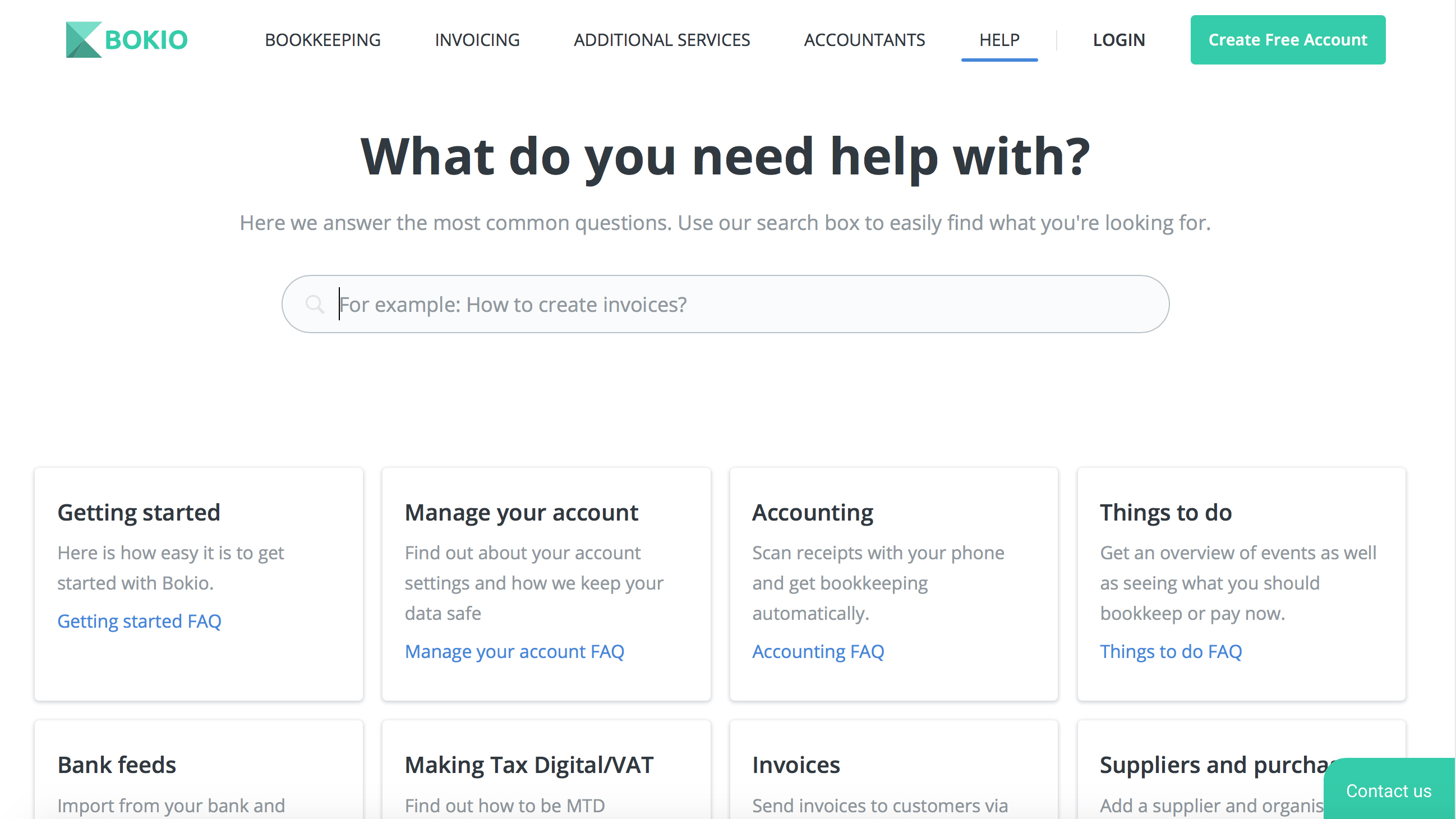The image depicts the landing page of the Bokeo platform, which prominently features a large search field in the center accompanied by the prompt, "What do you need help with?". The top main navigation bar, written in all caps with black text, includes options such as BOOKKEEPING, INVOICING, ADDITIONAL SERVICES, ACCOUNTANTS HELP, along with buttons for LOG IN and CREATE A FREE ACCOUNT, the latter being highlighted in a teal-colored button. The Bokeo logo also sports the same teal color.

Beneath the search field, various topics are listed, each within its own tile square. These topics include Getting Started, Managing Your Account, Things to Do, Bank Feeds, Making Tax Digital VAT, Invoices, Suppliers, and Purchases. There is also a 'Contact Us' button presented with a white background.

Additionally, a pop-up reveals statistics and information about user classifications. It notes that 10% of the average users classified as receiving a letter from a public institution and that 11% of restaurants and local businesses are restricted from removing pencils, even temporarily. The company behind this pop-up clarified that they are a corporate entity, not a restaurant, and are actively working with the town of Elk Grove to address this issue.

Thank you for reserving this conversation.